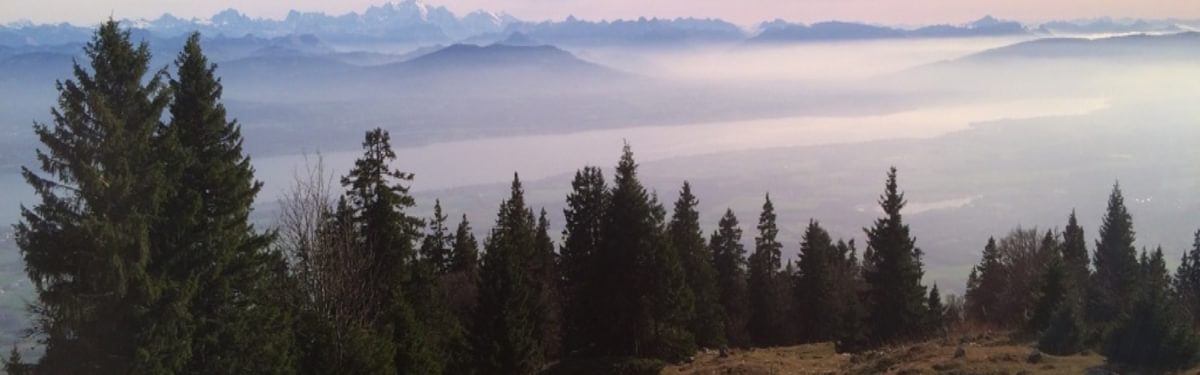A panoramic color photograph captures a breathtaking mountain landscape shrouded in mist, evoking the chill of a wintry or overcast day. In the foreground, a long row of towering conifer trees stands prominently, interspersed with a couple of deciduous trees. The trees vary in height, with the tallest on the left gradually getting shorter towards the right. The base of the trees is punctuated by a grassy, vegetated hillside. The distant mountains, possibly snowcapped, emerge through the hazy veil of mist and clouds that dominate the scene, giving them a whitish tinge. Additionally, a light-colored stream-like shape stretches from the left side of the photograph to the upper right, leading to ambiguity—is it a cloud or a river winding through the valley below? The sky above transitions through shades of blue, white, and touches of pink, reinforcing the scene's ethereal and serene quality.